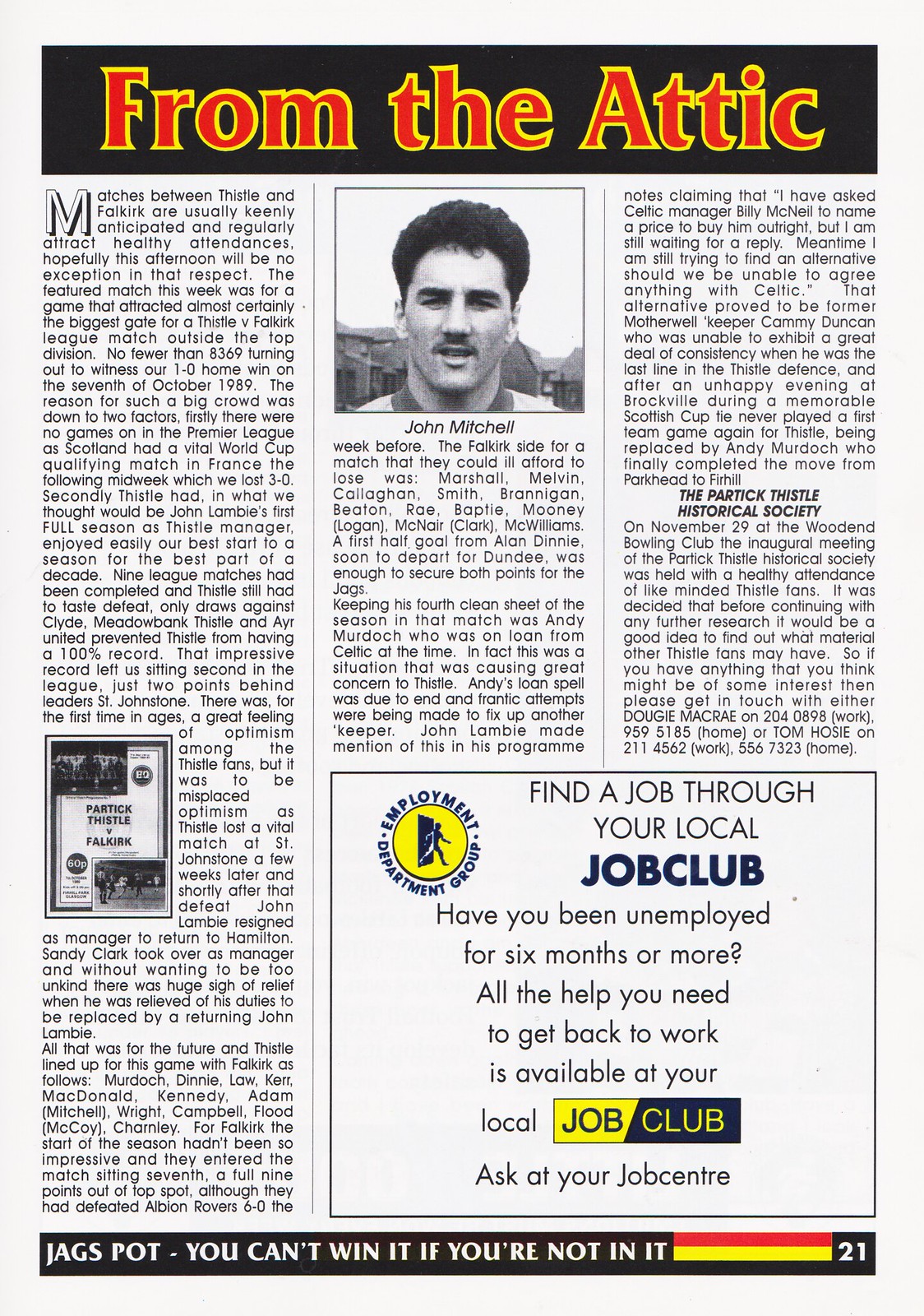This image portrays a page from a vintage publication, most likely a magazine, featuring detailed coverage of a historical football match between Partick Thistle and Falkirk. The page is predominantly white with a black header and a prominent red title outlined in yellow that reads "From the Attic." The text, arranged in multiple columns, passionately recounts a significant Thistle versus Falkirk game held on October 7, 1989, which drew an impressive crowd of 8,369 spectators due to two main reasons: no Premier League games on the same day and Thistle's strongest start to a season in a decade under manager John Lambie.

The narrative describes the teams’ lineups, Thistle’s solid defensive record led by on-loan Celtic goalkeeper Andy Murdoch, and the vital 1-0 victory secured by Allen Denny's first-half goal. The backdrop of Thistle’s temporary optimism, subsequent managerial shifts, and player transitions, including attempts to permanently acquire Murdoch, is vividly illustrated.

In the middle column stands a picture of a mustached John Mitchell, possibly a player or a coach, adding a personal element to the historical account. Adjacent to this, the bottom right corner contains a large advertisement promoting a job club for those unemployed for six months or more, emphasizing available assistance at local job centers. The page concludes with the phrase "Jagspot: You can't win it if you're not in it," and is identified as belonging to page 21.